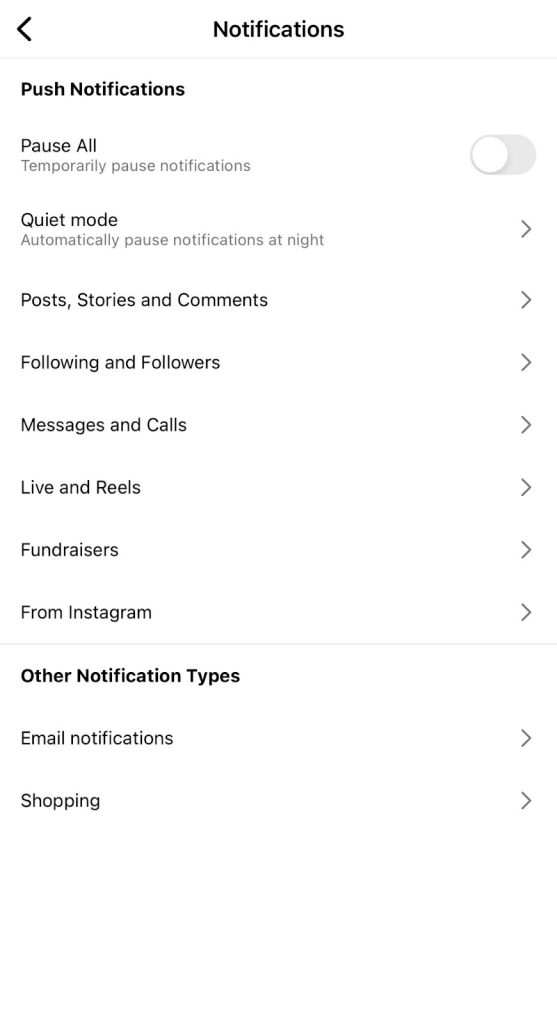The image displays a notification settings menu on a mobile phone. At the top left corner, a back arrow icon is visible, followed by the header text "Notifications." Below the header, a gray divider line separates it from the rest of the menu. 

The first bold, black text label reads "Push Notifications." Under this category, several options are listed:
1. **Pause All**: Includes a description "Temporarily Pause Notifications" with a toggle button shown as off.
2. **Quiet Mode**: Described as "Automatically Pause Notifications at Night," with a right-arrow indicating further settings accessible.
3. **Post Stories and Comments**: Includes a right-arrow indicating a submenu.
4. **Following and Followers**: Also has a right-arrow for additional settings.
5. **Messages and Calls**: Features a right-arrow for more options.
6. **Live and Reels**: Comes with a right-arrow for extra settings.
7. **Fundraisers from Instagram**: Has a right-arrow indicating more menu layers.

A second gray divider line further separates the next section titled "Other Notification Types." Under this section:
- **Email Notification**: Indicates more settings accessible via a right-arrow.
- **Shopping**: Also comes with a right-arrow leading to additional menus.

The purpose of this menu is to allow the user to customize which notifications to enable or disable on their mobile phone.